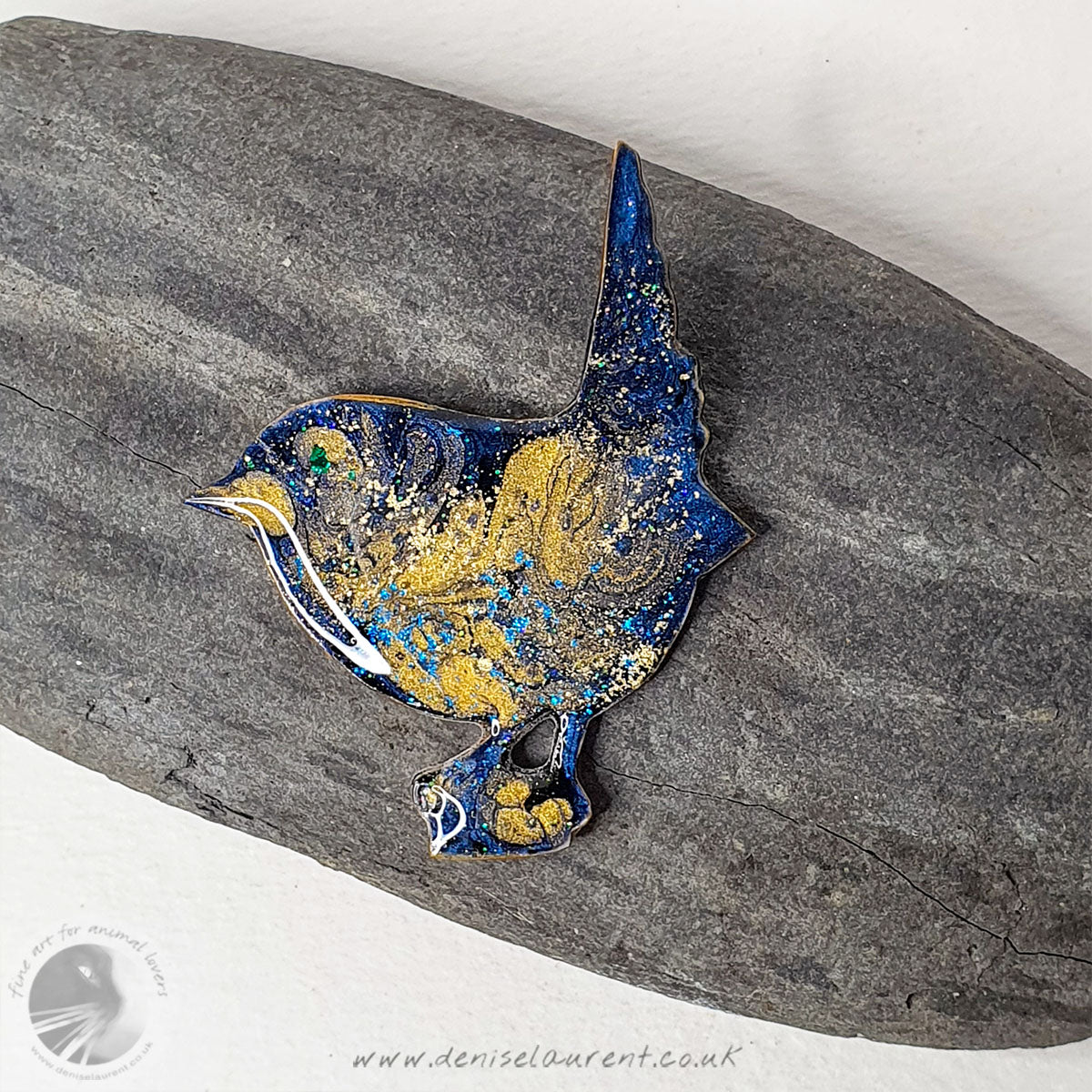This image features a decorative glass bluebird ornament, prominently positioned at the center and occupying about 25% of the frame. The bluebird, crafted from a glossy blue glass, showcases a yellow beak, green eyes, and additional yellow accents around the eyes and midsection. The tail is upright, and the legs merge seamlessly with the yellow detailing. The bluebird rests on a black or gray stone against a light gray background. There appears to be some debris or sand on the ornament. The bottom right corner of the image contains a watermark, reading www.deniselaurent.co.uk, alongside a grayed-out circle emblem with the silhouette of a cat's head and the words "Fine Art for Animal Lovers."